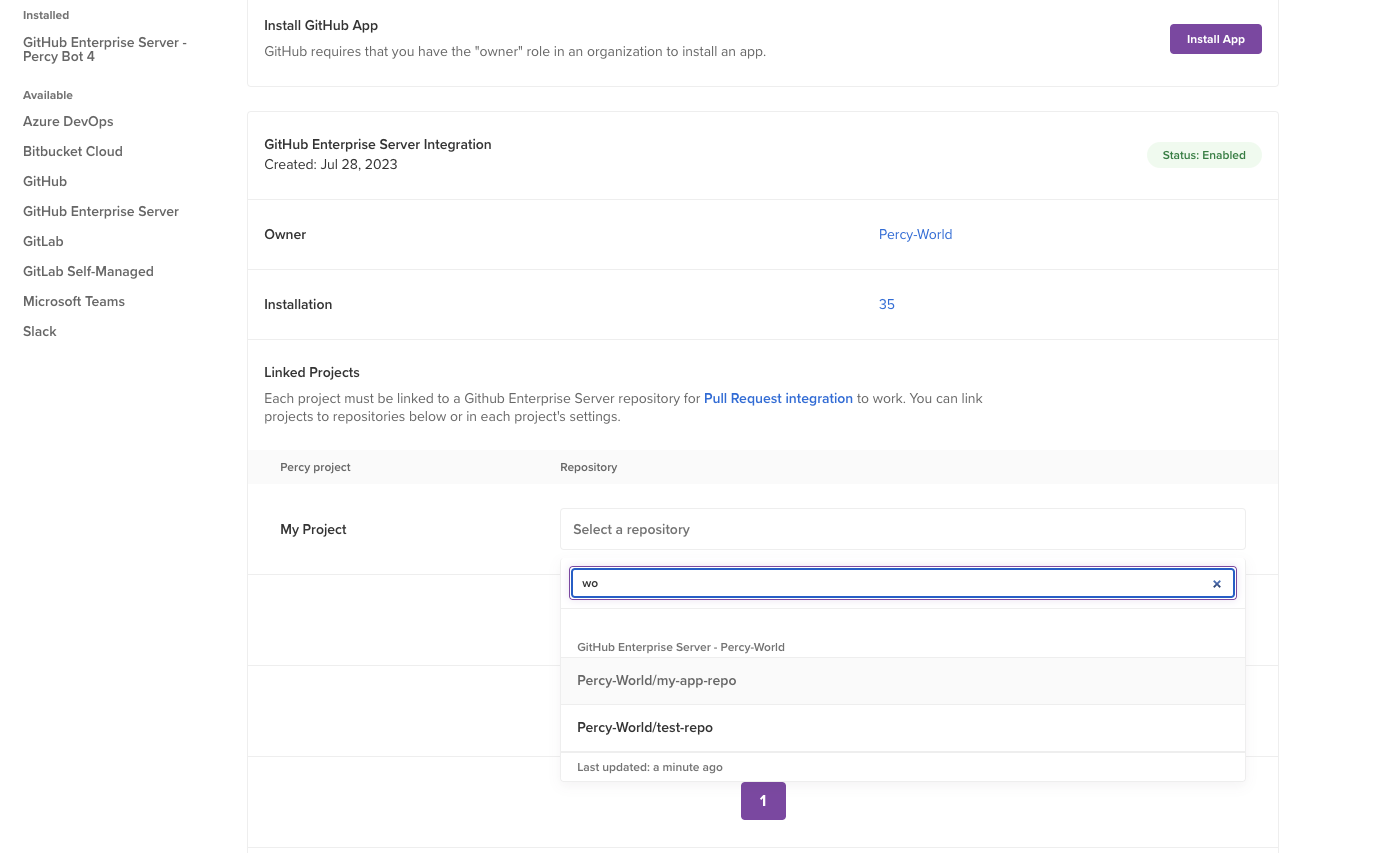The image displays a webpage interface for GitHub app integration. On the right side, there is a vertical menu with 11 options listed. The website features a predominantly white background. The menu to the left includes options for:

1. Installed GitHub Apps
2. GitHub Enterprise Server
3. Available Azure DevOps
4. Bitbucket Cloud
5. GitHub
6. GitHub Enterprise Server (listed again)
7. GitLab
8. GitLab Self-Managed
9. Microsoft Teams
10. Slack

The main content area primarily focuses on the installation of the GitHub app. There is a prominent purple button on the right side for app installation. The description beneath it indicates the requirement for an "owner" role within an organization to install the app.

Below this description, there is a section dedicated to GitHub Enterprise Server integration, highlighted by a green tab that reads "Status: Enabled." The section notes that the owner is "Percy World," with the installation count listed as 35. There is also a linked project area named "My Project," where users can select a repository.